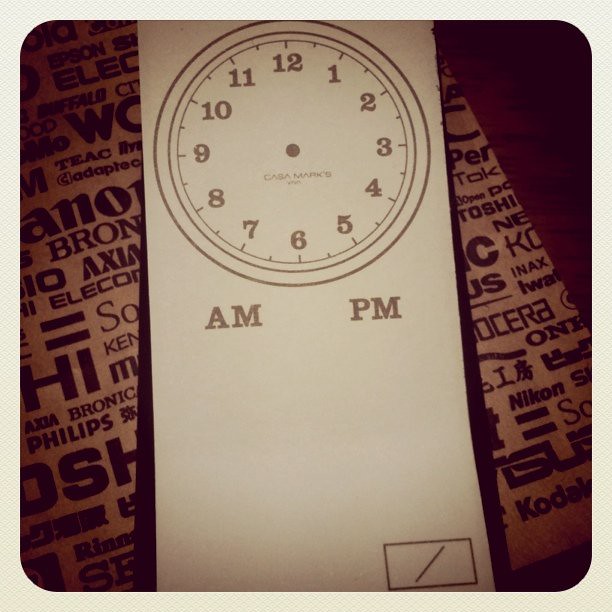The photograph captures a detailed, round clock, embossed in black on a stark white sheet of material. The clock features black numbers on a white clock face and prominently displays the letters "AM" and "PM" in bold black text beneath it. At the bottom center of the white material, there is a distinctive rectangle housing a black slash mark. This white sheet with the clock is resting on top of what appears to be a paper insert, which is also white and covered in various black brand names such as Nikon, Philips, and Kodak, among others. The entire image is characterized by an overexposed, brightly washed-out lighting effect, lending it a high-key, ethereal aesthetic.